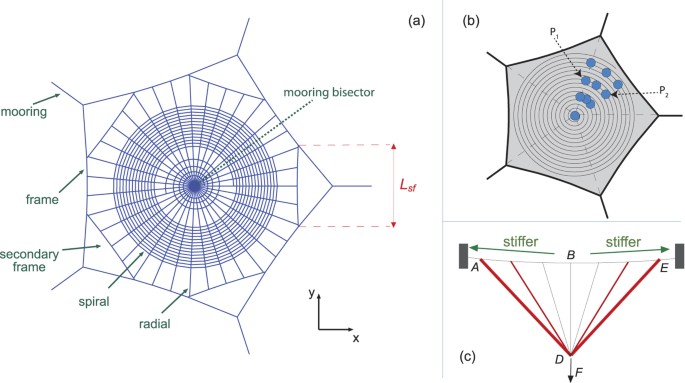The diagram is divided into three main sections. On the left side, the image features a complex spider web-like structure, characterized by its hexagonal or octagonal shape. This structure is illustrated in dark blue, with multiple lines and circles radiating from its five corners towards the center, forming an intricate network. These lines and circles are annotated with green lettering and dotted arrows indicating various design elements such as "mooring bisector," "frame," "secondary frame," "spiral," and "radial."

To the right, the diagram is split into two subsections labeled B at the top and C at the bottom. Subsection B showcases a similar spider web-like design as the main image, with blue circles and additional annotations. Subsection C, located below, features a V-shaped pattern highlighted in red and blue, with arrows pointing to the structure marked as "stiffer." Both subsections are interconnected by arrows and letters, including C, A, B, E, D, and F, providing further details on the diagrams’ components and their relationships, with a clear emphasis on structural stiffness and design mechanics. Additionally, a formula labeled LSF is noted, emphasizing the diagram's analytical nature.